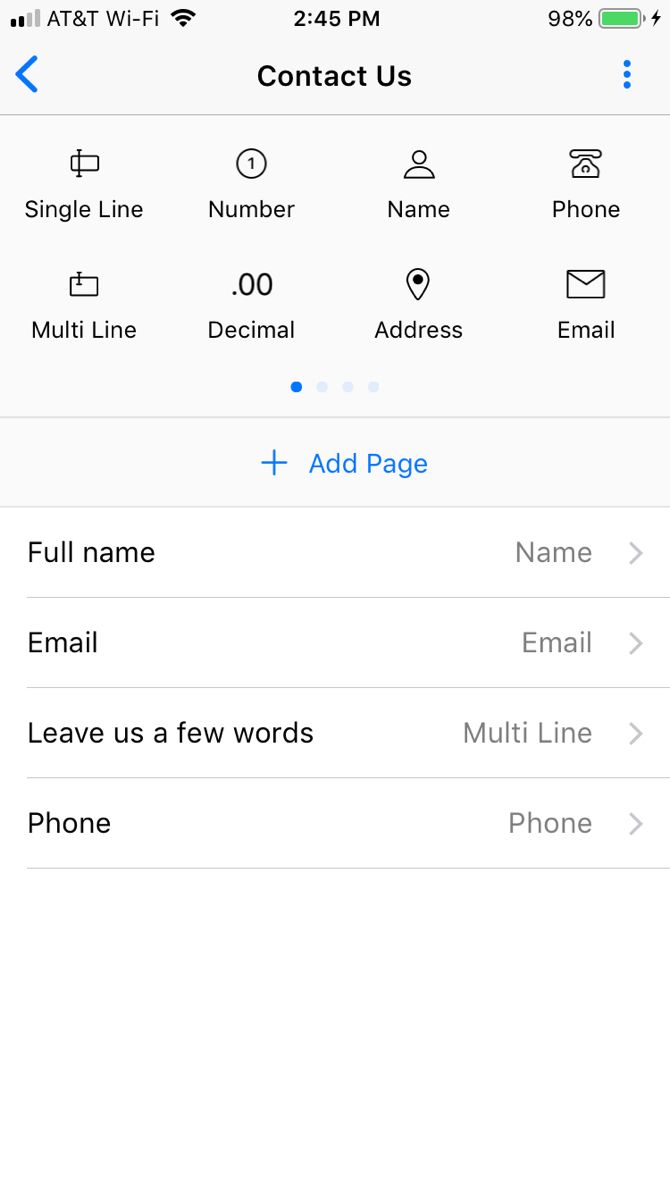A screenshot of a user's cell phone interface taken at 2:45 p.m. with 98% battery life, connected to AT&T Wi-Fi. At the top-left corner, the Wi-Fi signal icon and the current time are displayed. Adjacent to those indicators, at the center of the screen, the text "Contact Us" is visible. A blue left-pointing arrow is situated to the left of "Contact Us," and on the right, there is a vertical column of three blue dots, likely representing additional menu options. Below this header, there is a list of form fields, including "single line," "number," "name," "phone," "multi-line," "decimal," "address," "e-mail," "add page," "full name," "name," "e-mail," "leave us a few words," "multi-line," "phone," and "phone." The screenshot is of a portrait orientation, resulting in an image format taller than it is wide. The image does not contain any people, animals, birds, fish, plants, flowers, trees, signs, billboards, flags, banners, buildings, man-made structures, airplanes, or automobiles.